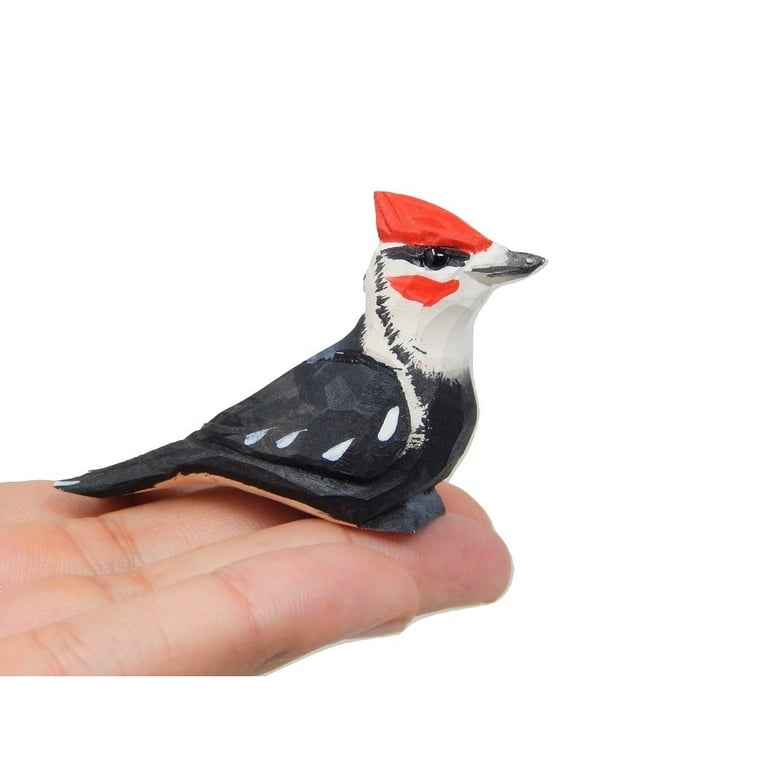The image features a small, hand-painted wooden bird figurine resting on the four outstretched fingers of an unseen person's hand against a completely white background. The bird, positioned facing to the right, appears to be a folk-art rendition resembling a woodpecker. Its head is primarily white with a striking red top notch and a red patch under its eye. The beak is a subtle gray, not fully black. Distinctive black markings encircle its eye and run from the back of the head down to the front of the chest. The bird's body is predominantly black, adorned with about four white spots on the wings, a touch of white on the underside of the body visible from this angle, and a hint of white on the tail. The figurine, amateurish and child-like in its construction, likely stands between 2 to 3 inches (approximately 5 to 7.5 cm) tall. The visible left hand holding the bird is palm up, offering a clear view of the bird perched delicately on the fingertips.